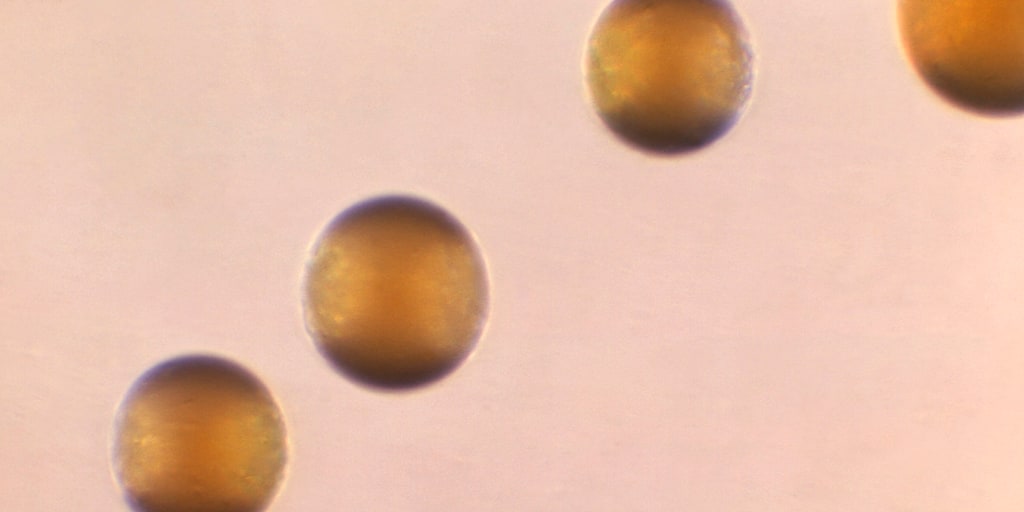This abstract image, reminiscent of a 1970s magazine photograph, features a grainy, vintage aesthetic. Set against a salmon pink background are four amber-colored circles. These circles have areas of black discoloration at the top and bottom, giving them a slightly translucent appearance in places. The overall composition is minimalistic, with no other objects, text, or elements present, allowing the circles to stand out prominently. The image's fuzzy, nostalgic quality enhances its retro feel, making for a visually intriguing piece.